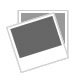This color photograph showcases the packaging for a Hamilton Beach Stand Mixer, prominently featuring a white box with bold black text at the top that reads "Hamilton Beach." Beneath this, the text "Stand Mixer" is displayed, along with a blue circle bearing the phrase "Same mixing action as KitchenAid stand mixers." The image of the mixer itself reveals a predominantly white or silver body with black accents, including a handle on top and knobs on the side. It highlights the powerful 300-watt motor and complete bowl coverage mixing action, depicted with arrows. Detailed text on the box promotes its superior mixing compared to two-beater stand mixers, listing features such as three attachments for mixing versatility, a four-quart stainless steel bowl with handles, an included splatter shield, and seven adjustable speeds. The bottom right corner of the box shows images of included accessories: a dough hook, whisk, and flat beater. The mixer appears to be situated on a tiled kitchen counter, adding a realistic touch to the packaging presentation.